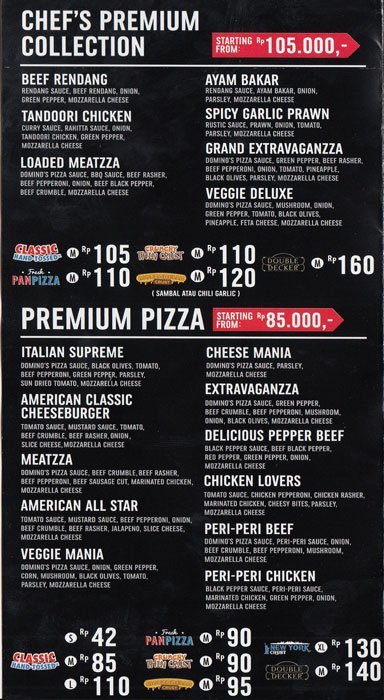The image portrays a restaurant menu with a sleek black background, segmented into two prominent sections. The top section is labeled "Chef's Premium Collection" in bold white text, featuring detailed descriptions of an array of dishes. This section lists sophisticated culinary offerings such as Beef Rendang with Rendering Sauce, Tandoori Chicken in Curry Sauce and Ranita Sauce, and Loaded Mitsu with Domino's Pizza Sauce and Barbecue Sauce, complemented by ingredients like onion, green pepper, and mozzarella cheese. The second column extends the collection with dishes like Ayam Bakar paired with Randag Sauce, garnished with onion and parsley.

Beneath the "Chef's Premium Collection," the menu continues, though the text becomes more condensed and harder to discern. Highlighted in this section are premium pizzas. These pizzas include intriguing combinations like Spicy Garlic Prawn, Ground Extravaganza, Veggie Deluxe, Italian Supreme, and American Classic Cheeseburger, with prices starting from 85.000. The visually striking menu balances its black backdrop with various text colors, featuring blues, browns, reds, and whites, creating a vibrant yet elegant display centered on the page, resembling the layout of a large cheese stick at both the top and bottom of the menu. 

Overall, the menu's design suggests an upscale dining experience, emphasizing gourmet dishes and premium pizzas with meticulous detail and an inviting presentation.